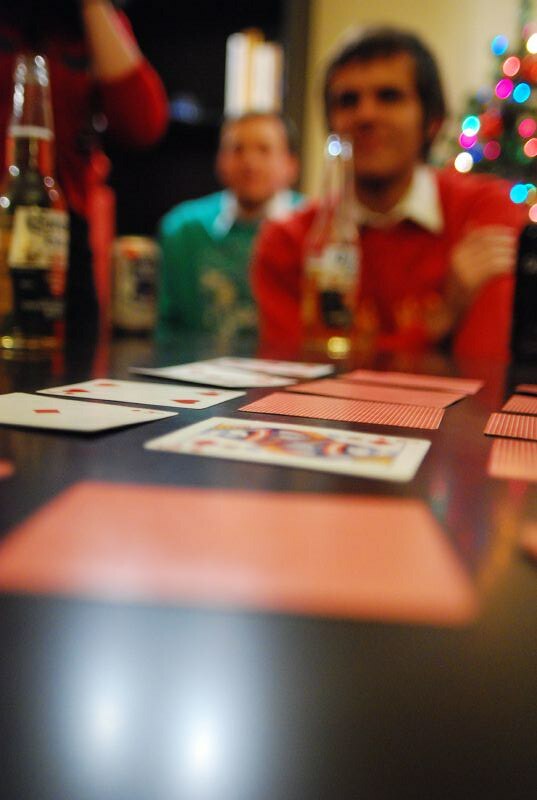The image is a fuzzy, out-of-focus color photo likely taken during Christmas time, suggested by the multi-color twinkling lights on a tree shape visible in the top right corner. The main subject of the photo is a glossy-surfaced table, glaringly reflecting bright white lights in the bottom left. Arranged on this glossy table are several playing cards, some face up and some face down, which possibly indicate someone is engaged in a game of solitaire or a memory card game. The face-up cards include a Queen of Hearts or Diamonds, an Ace of Diamonds, and a 4 of Hearts or Diamonds, while the face-down cards have a red and white pattern. 

Facing the camera is a man wearing a festive red sweater, presumably an ugly Christmas sweater, over a white collared shirt. He has long hair and a half-drunk clear glass bottle of what appears to be Corona beer in front of him. Behind his right shoulder, toward the upper left of the photo, sits another man in a green sweater with a collared shirt. Partially visible on the upper left is a third person, dressed in red but cropped to reveal only their forearm and torso. Another larger bottle of Corona beer is closer to the camera, along with a can of Pabst Blue Ribbon beer further back on the table. In the background, a window lets in some light, while the backdrop seems to be a dark wall. The scene captures a casual, festive atmosphere with elements of holiday cheer and leisure.